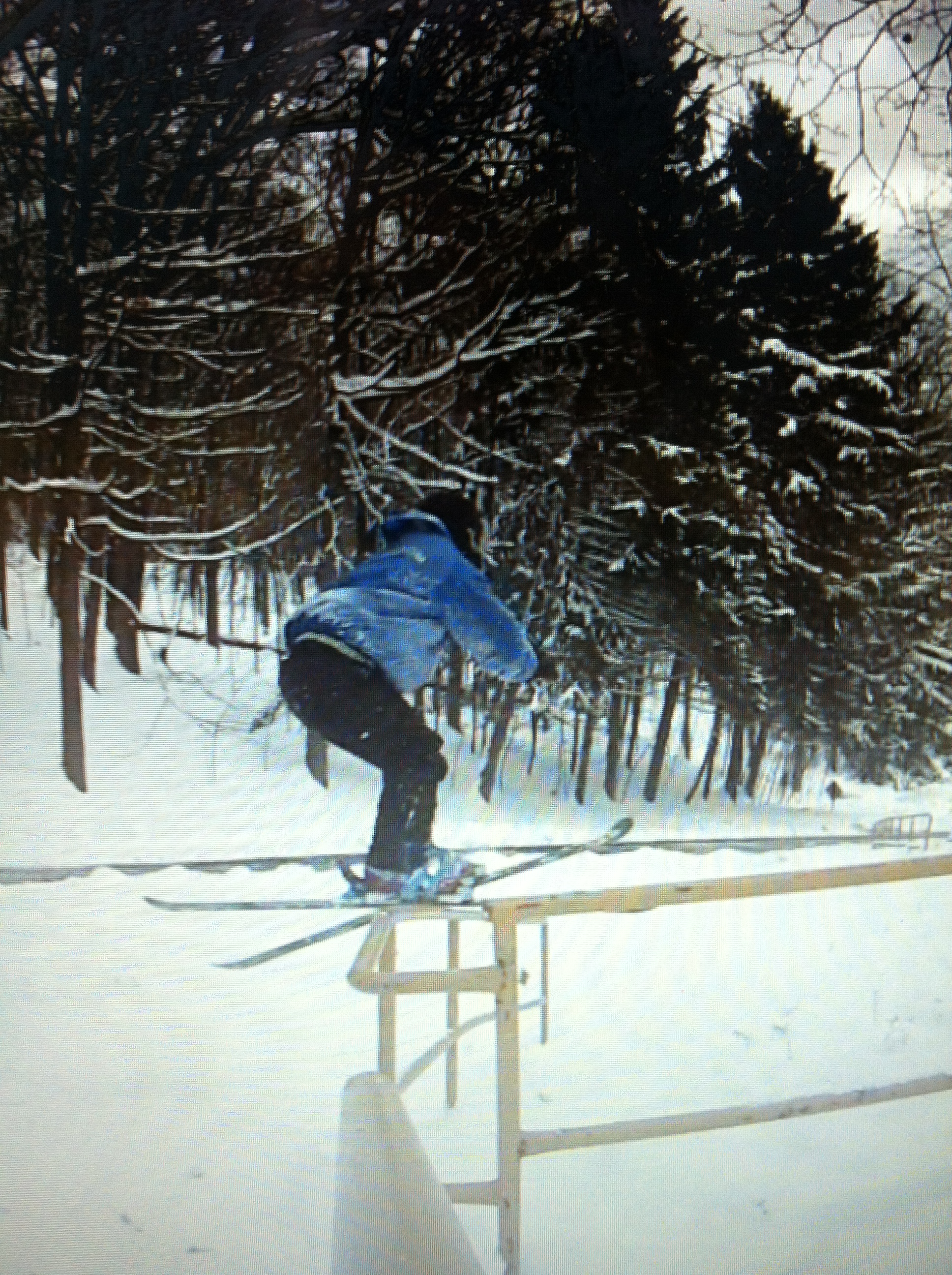This slightly blurry outdoor winter scene, likely taken with a personal or cell phone camera, captures a thrilling ski stunt. The focal point is a skier in a blue jacket and black pants, perched precariously atop a beige-colored metal rail, perhaps intended to prevent passage. The skier’s blue bindings are visible as they balance or grind along the rail, reminiscent of a skateboarder on a grind. This dramatic action appears set at a ski resort or hill and is surrounded by a snowy landscape with evergreen trees heavily laden with snow in the slightly distant background. The overcast, cloudy sky adds to the ambiance of this snowy day. The ground beneath is completely covered in snow, with a groomed ski trail visible to the left of the skier. There’s a light wood or mesh fence in the foreground, contributing to the scene’s depth and the skier’s daring stunt.